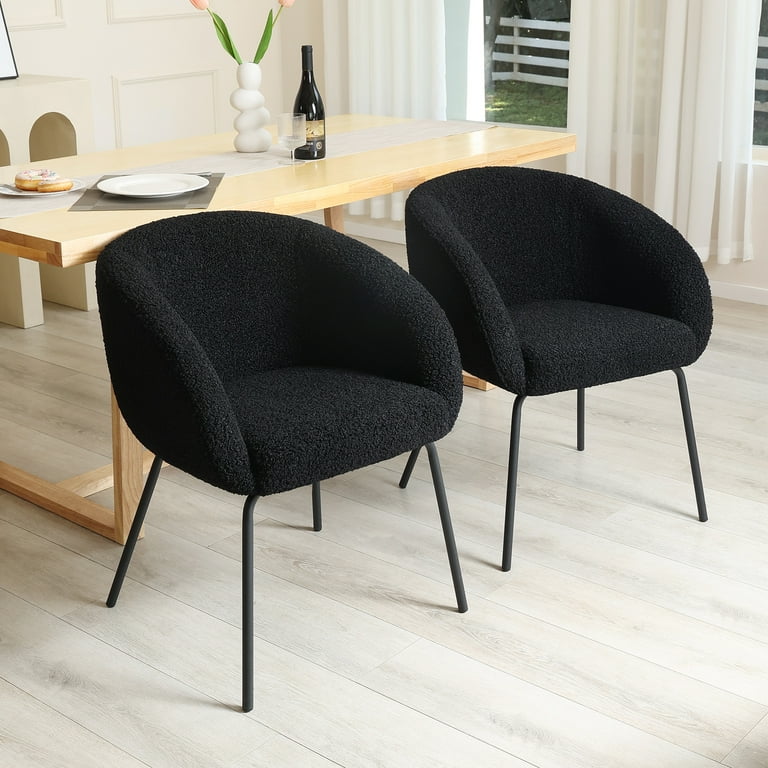This is a detailed photograph of a residential interior featuring two identical, modern, mid-century modern black chairs. The chairs are upholstered in a fuzzy, felt-like material, with a seamless armrest-to-backrest design that curves smoothly down towards the seat cushion. Each chair is supported by slender, black pin legs and reaches about mid-back height. They are positioned next to a light brown wooden table adorned with various items: a bottle of wine, an empty wine glass, a vase resembling stacked rocks containing two pink flowers with green stems, a gray placemat with a white plate, and another white plate with a donut. A light gray table runner stretches across the table. The room is decorated with white wainscot paneling on the walls, and the floor is covered in pale white hardwood. In the background, there is a large window framed by long white curtains, through which a well-manicured grass lawn and a white fence are visible, completing the serene and modern ambiance of the room.